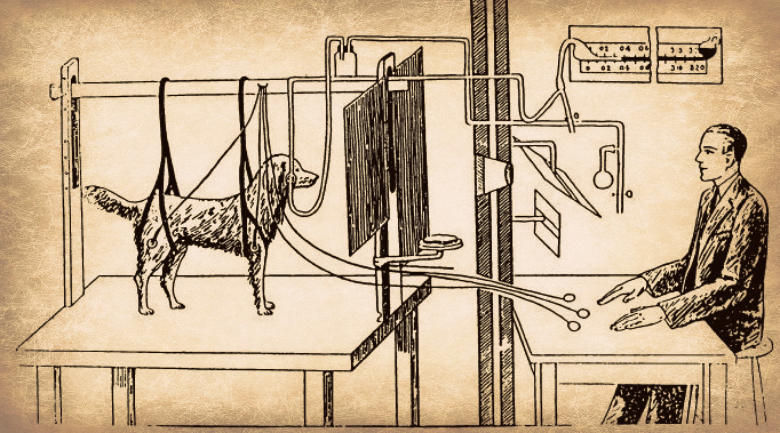This black-and-white comic illustration depicts a surreal laboratory setting featuring a man and a dog facing each other across separate tables. On the left side, there is a medium-sized dog standing on a table, restrained by numerous harnesses around its back and front legs. The dog is connected to several wires and tubes, one of which extends near its jaw. A black screen hinders its vision, adding to the sense of experimentation. In the center, two vertical black lines serve as a partition between the dog and the man. The man, located on the right side, is dressed in a black business suit and tie, and is seated on a stool at a different table. He rests his hands palms down on the table, where three buttons are positioned in front of him. The background features various measurement charts, meters, and apparatuses, contributing to the scientific ambiance of the scene. The overall illustration is rendered on aged, yellowed paper, adding an antique, dated feel to the image.